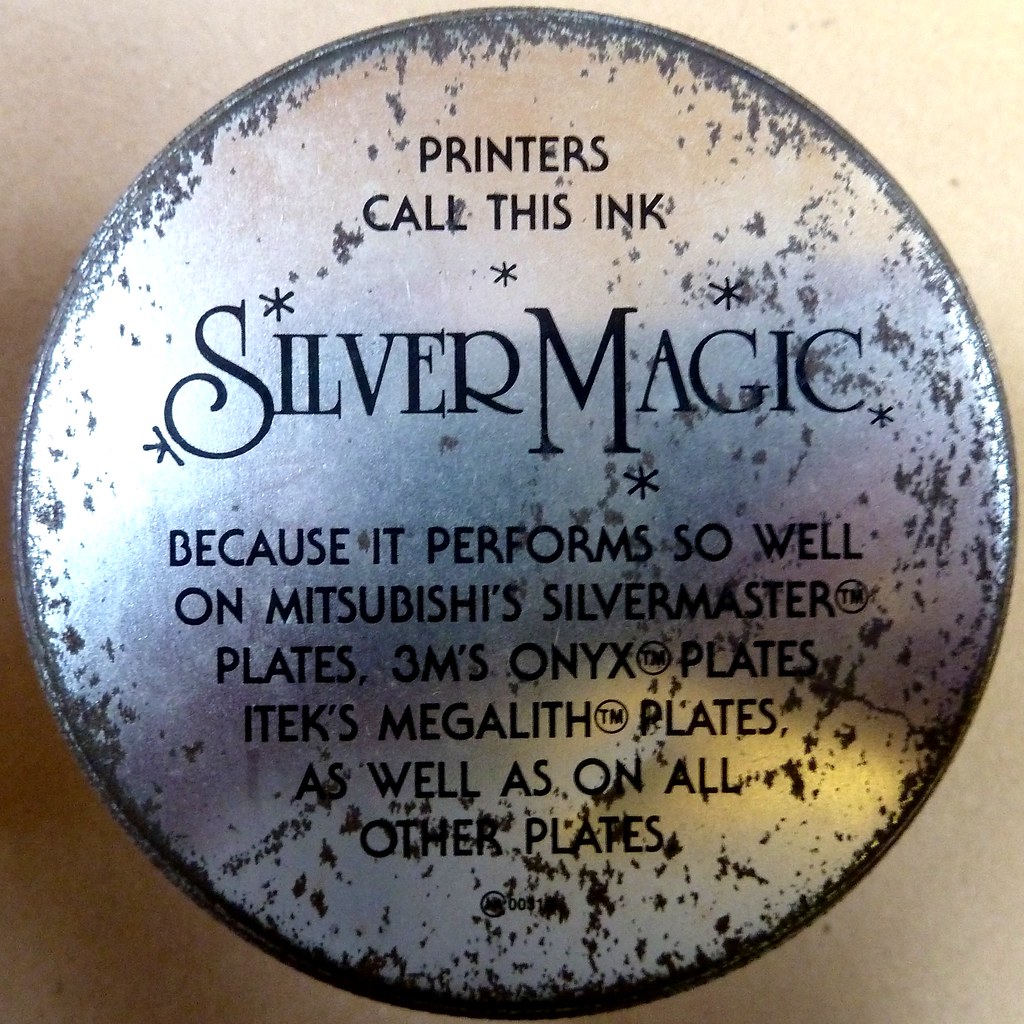The square image prominently features a large, tarnished silver disc that extends to the edges of the frame. The silver surface, which appears aged and worn, particularly around the edges, reveals areas where the luster has faded to a darker gray, and there are black patches suggesting either rust or chipped paint. The disc contains black printed text, with the headline “Printers call this ink” placed above the center. Below this, in significantly larger and more elaborate font, the words “Silver Magic” stand out. Underneath that, in smaller print, the text reads, “Because it performs so well on Mitsubishi’s Silver Master plates, 3M’s Onyx plates, Itek’s Megalith plates, as well as on all other plates.” Tiny asterisks are sprinkled around the image, adding to the intricate detail. The subtle background behind the metal object is a light beige or brown, blending seamlessly with the metallic appearance.